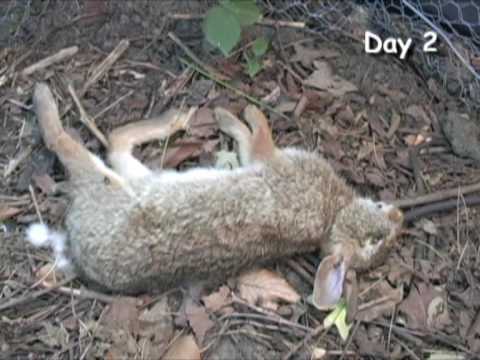In this poignant photograph, a dead jackrabbit lies on its side, upside down, on a forest floor scattered with dirt, dried leaves, and broken branches. The rabbit's natural fur colors—brown and gray—are visible, and its white fluffy tail is noticeable near its rear end. Its back is turned towards the viewer, with its legs sticking out; the two back legs extended and the front paws shorter, one resting on top of the other. The rabbit's eyes appear to be open, albeit possibly just a slit. A small patch of green leaves is seen at the top center of the image, adding a minor touch of life to the otherwise somber scene. There’s text in the top right corner that reads "Day 2," suggesting that this photograph is part of a series documenting the decay of the carcass. The overall atmosphere of the image is sad, emphasizing the stark stillness of the forest in contrast to the once vibrant life of the rabbit.